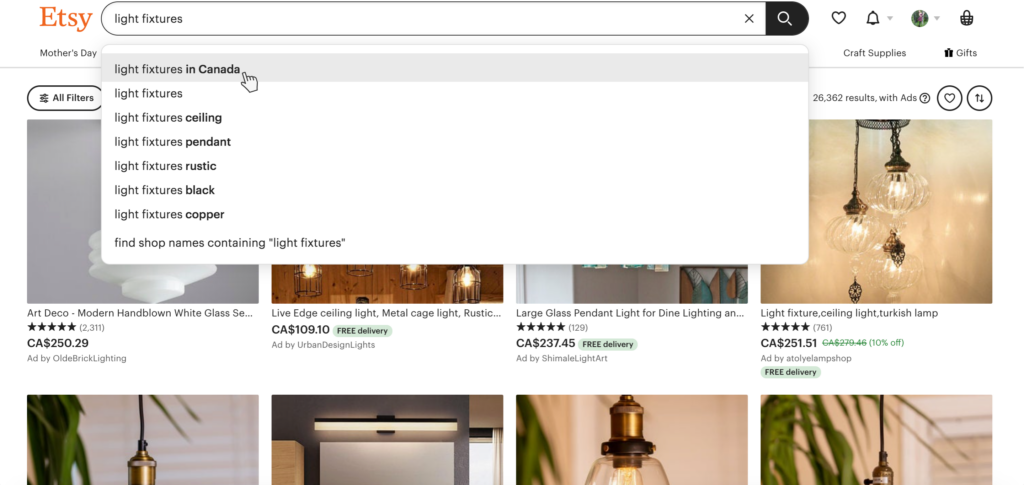This is a detailed caption for an image, based on an elaborate description provided via voice, of a user account screenshot from the Etsy marketplace. 

---

Screenshot of an Etsy Marketplace User Account Interface:
 
At the top center of the screenshot, the recognizable orange "Etsy" logo is prominently displayed, doubling as both text and logo. Just beneath the logo, there's a visible category titled "Mother's Day," while other category options remain hidden. Adjacent to this, a large, horizontal search bar is noticeably present, equipped with a magnifying glass icon for searching, an "X" for clearing the search text, and the placeholder text "light fixtures" indicating the current search input.

The smart search bar has offered a dropdown menu listing various related search suggestions: "light fixtures in Canada" (being selected by a cursor), followed by "light fixtures", "light fixtures ceilings", "light fixtures pendant", "light fixtures rustic", "light fixtures black", and "light fixtures copper". There is an additional option, "wine shop names containing light fixtures," showcasing its comprehensive search capability.

To the right of the search bar, there are icons representing a heart for favorites, a bell for notifications, the user profile, and a shopping basket, reflecting a typical e-commerce layout.

Beneath the search bar, a category titled "Craft Supplies and Gifts" is highlighted. The main portion of the screen advertises various light fixtures in distinct styles, showcasing product thumbnails, review ratings, and cover images, providing the user a glimpse into the products available for purchase within the category.